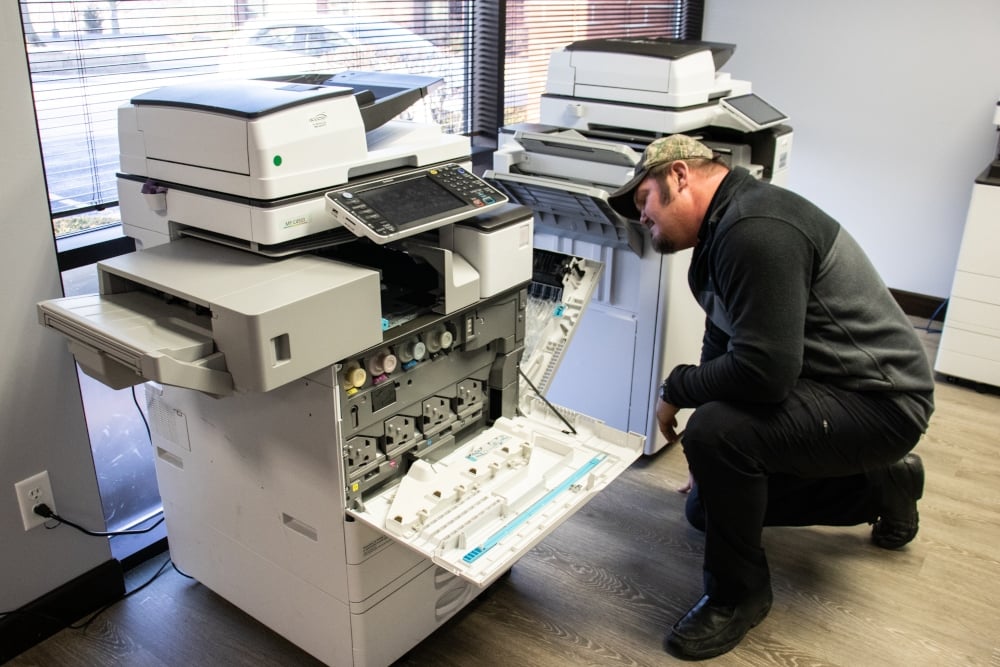In this color landscape photograph, a man is kneeling on one knee on the hardwood floor of an office-like environment, deeply absorbed in inspecting the open interior of a large copier machine. Situated in front of a floor-to-ceiling window with raised blinds, the scene glimpses a parking lot outside. The man, appearing to examine possible mechanical issues, is wearing a camouflage hat, a black and gray jacket with black sleeves, black pants, and black shoes. He has a pale complexion and a goatee. The copier machine, which has its front covers open and a tablet-like touchscreen interface, stands prominently in the middle. To the right of this machine, another similar copier is partially visible, emphasizing the typical office setting. The bright, white walls and the clear view of the equipment's intricate interior parts, knobs, and dials, as well as the outlet it is plugged into, contribute to the realistic, representational style of the photograph, capturing a moment of detailed, technical focus.